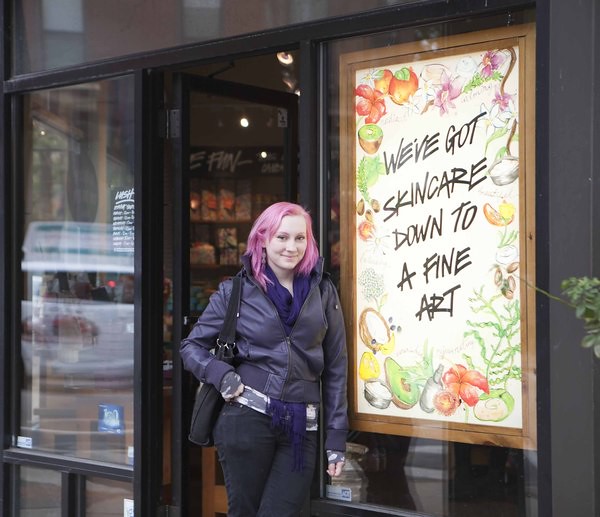A vibrant, square-cropped color photograph features a smiling woman with short, bright pink hair and fair skin standing centrally in front of a store. She dons a purple scarf tucked into a purple zip-up leather jacket and black fingerless gloves, while a black purse hangs over her right shoulder. Her right arm is propped on her hip and her left arm hangs by her side. She wears form-fitting black jeans with a glimpse of a gray and white shirt underneath her jacket.

Behind her, the store has sleek black paneling and large glass windows reflecting the bright, clear midday. The storefront is adorned with a large, brown wooden-framed sign prominently displaying in black text, "We've got skin care down to a fine art," surrounded by illustrated fruits and vegetables like avocados, tomatoes, and kiwis. The store's interior is vaguely visible through the windows, showcasing neatly arranged shelves filled with various products, hinting at a beauty or skincare shop. A small green plant peeks from the right side of the frame, adding a touch of nature to the urban scene.